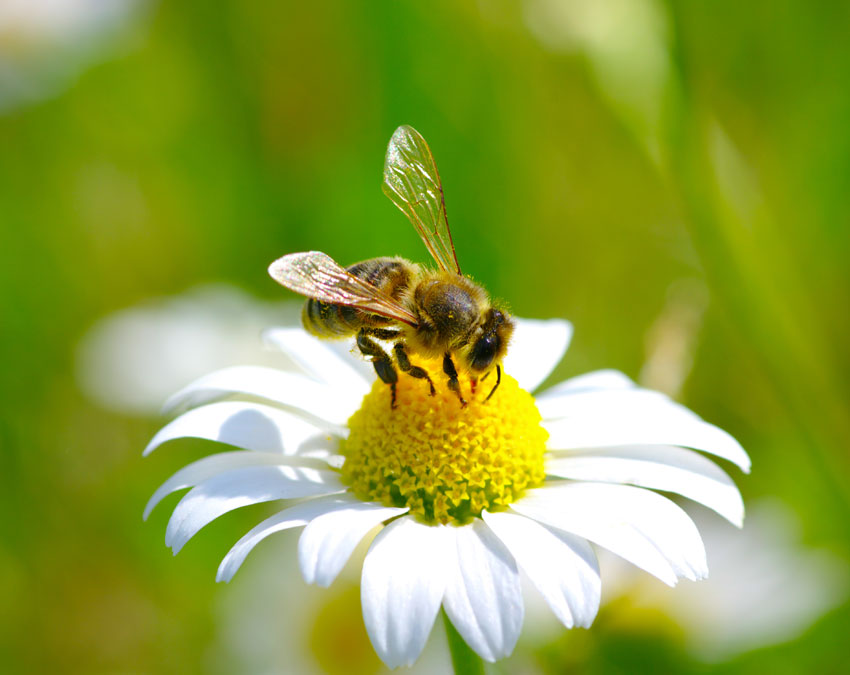This is a close-up, detailed photograph of a honey bee diligently gathering nectar from the center of a white daisy. The photo, captured outdoors during daylight, showcases the bee in a natural setting. The white petals of the daisy elegantly curve outward and slightly dip downward, encircling a vibrant yellow center that is composed of numerous tiny yellow florets. The background is beautifully blurred, creating a soft green bokeh effect that highlights the intricate details of the bee and the flower.

The honey bee, with its two transparent wings, has a distinct, hairy body adorned with yellow and gold fibers. The wings, positioned above its back, catch the light, making their translucence evident. The bee’s segmented body—particularly its head and claws—are embedded deeply in the flower’s center, as it works to extract the sweetness. The image captures the bee facing to the right, exhibiting its systematic method of nectar collection. The precise focus on the daisy and the bee, contrasted with the blurred background, brings an artistic and almost ethereal quality to this nature photograph.